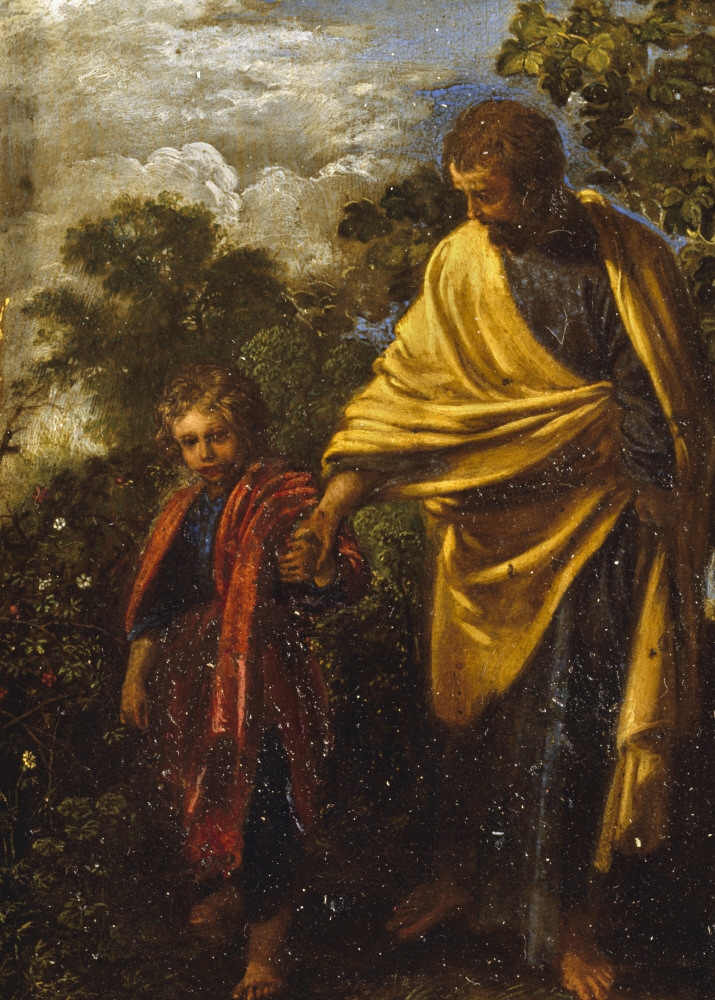This oil painting, exhibiting noticeable wear and tear with chipping and flaking, likely from the Renaissance era, features a barefoot man and a boy walking through a wooded area. On the right side of the image, the bearded man with brown hair is clothed in a gold or yellowish shroud over a dark undergarment that extends to his ankles. He holds the hand of the shorter boy standing to his left. The boy, who has blonde hair, wears a reddish shroud over a similar dark outfit. They seem to be walking amidst floral and vegetal elements, with flowers and trees surrounding them. The background depicts white clouds and patches of blue sky, suggesting it is daytime. The man gazes down at the boy, who looks towards the ground.